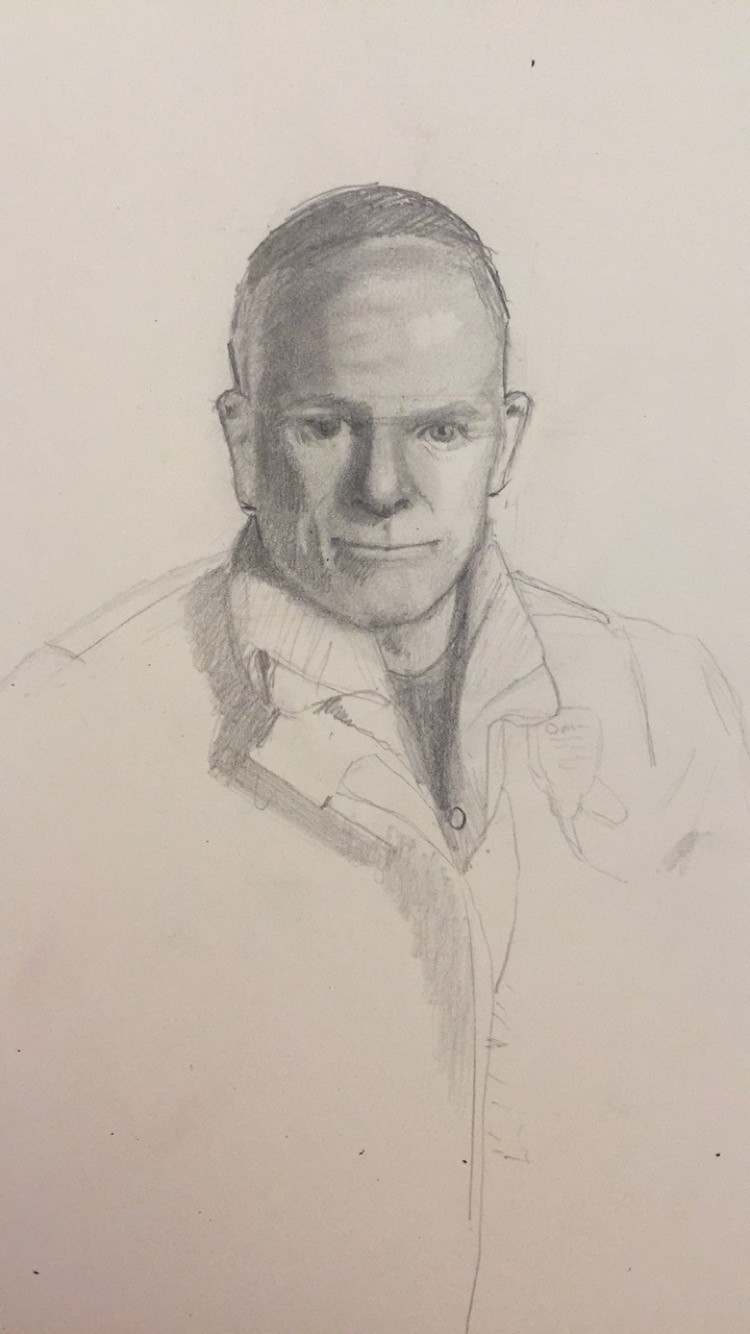The image features an incomplete pencil sketch of a middle-aged man. The fully detailed and shaded head and face contrast sharply with the lightly sketched and unfinished shoulders and torso. His hair, possibly combed to the side or resembling a short cap, appears darker on top, while the sides are left white, suggesting either a receding hairline or a distinct head covering. The man wears a coat with a large collar, sketched lightly with few details, and a dark-colored t-shirt beneath it. Though the coat seems to be buttoned, the specifics are unclear, but hints of button links are noticeable. The portrait’s meticulous shading on the face creates a three-dimensional effect, with one eye particularly detailed to show the pupil and the other rendered completely black. The nuanced shading and blending on his face and hair highlight the artist's focus on these areas, leaving the rest comparatively sparse.